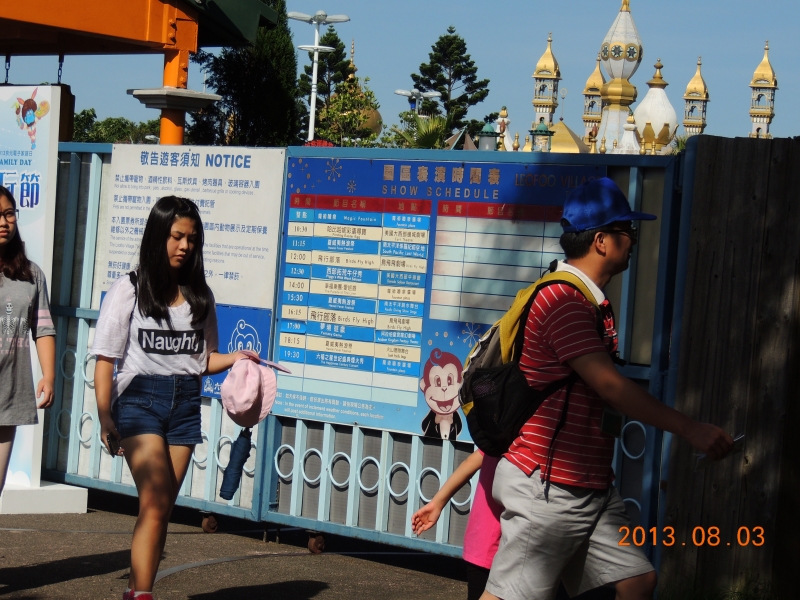The image, dated August 3, 2013, captures a sunny day with a clear blue sky at what appears to be a Chinese amusement park, possibly resembling Disneyland. Dominating the background in the upper right-hand corner is an ornate, gold and white castle-type structure with several towers and pillars, surrounded by tall green trees. In the foreground, several people are seen walking in front of a gated area adorned with banners and notices, some of which include Mandarin characters and an English "show schedule" sign.

To the left, a partially visible woman with glasses and long black hair, dressed in a gray t-shirt, appears alongside another woman in short jean shorts, a white t-shirt reading "Naughty," and long straight black hair. She holds a phone, a hat, and an umbrella in her left hand. Nearby, a man wearing a striped red and white shirt, khaki shorts, and a blue ball cap is pushing a stroller, accompanied by a small child in a pink shirt. Another young couple, dressed in summer clothing, appears on the right side of the image, also making their way towards the entrance. The scene is lively, with families and friends enjoying an outing under the bright sun.